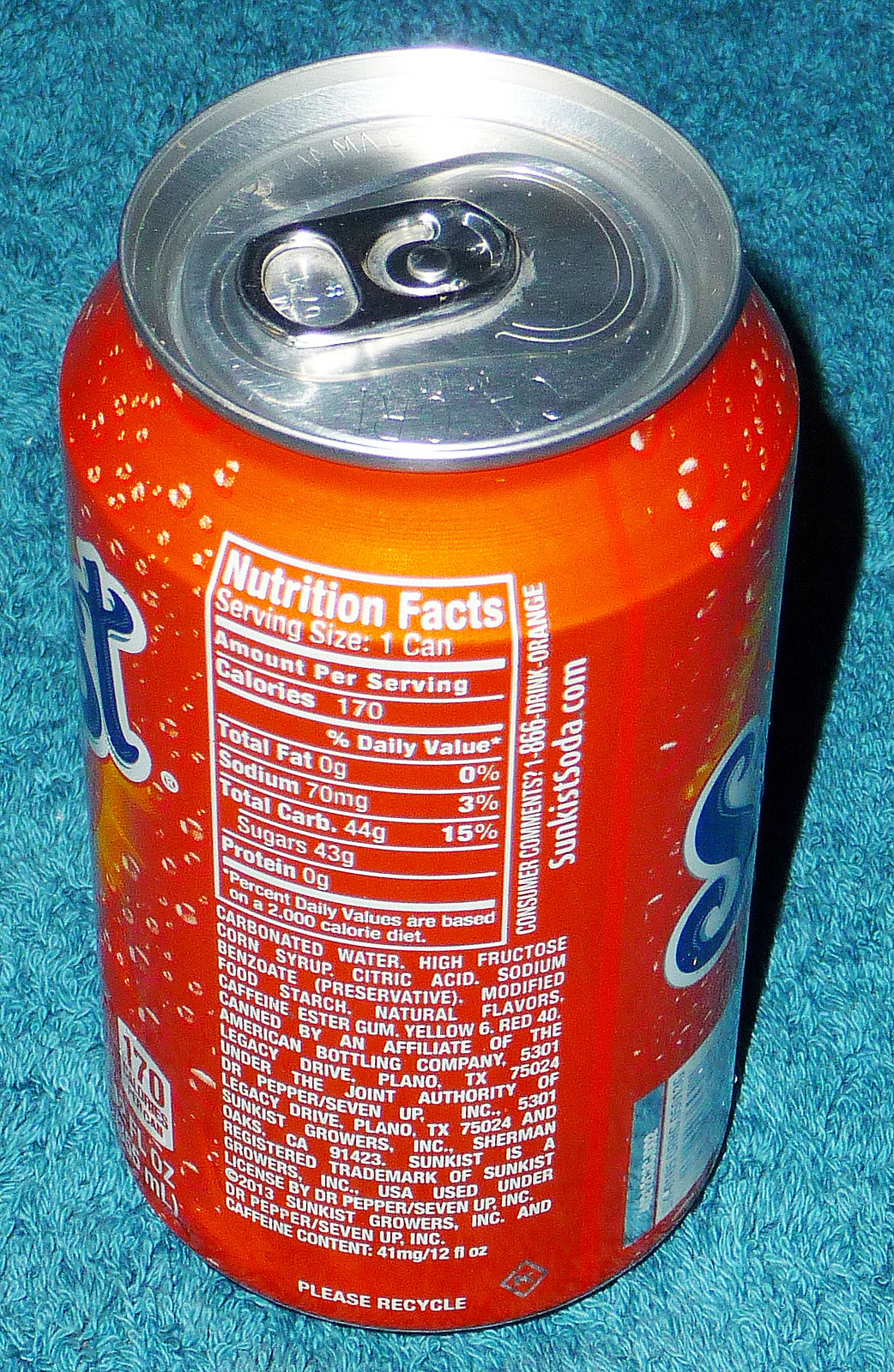This close-up photograph captures an orange Sunkist soda can prominently displaying its nutrition facts label. The can, with its silver aluminum top and distinctive pop tab, sits on what appears to be a blue textured fabric. The focal point is the white nutrition label, which details the serving size of one can, 170 calories, 70 milligrams of sodium, and 43 grams of sugar, among other nutritional information. Ingredients listed include carbonated water and high fructose corn syrup. The can also features messages such as "Please Recycle" along with the recyclable logo. The sides of the can partially reveal the letters 'S' and 'T', further indicating the Sunkist brand.